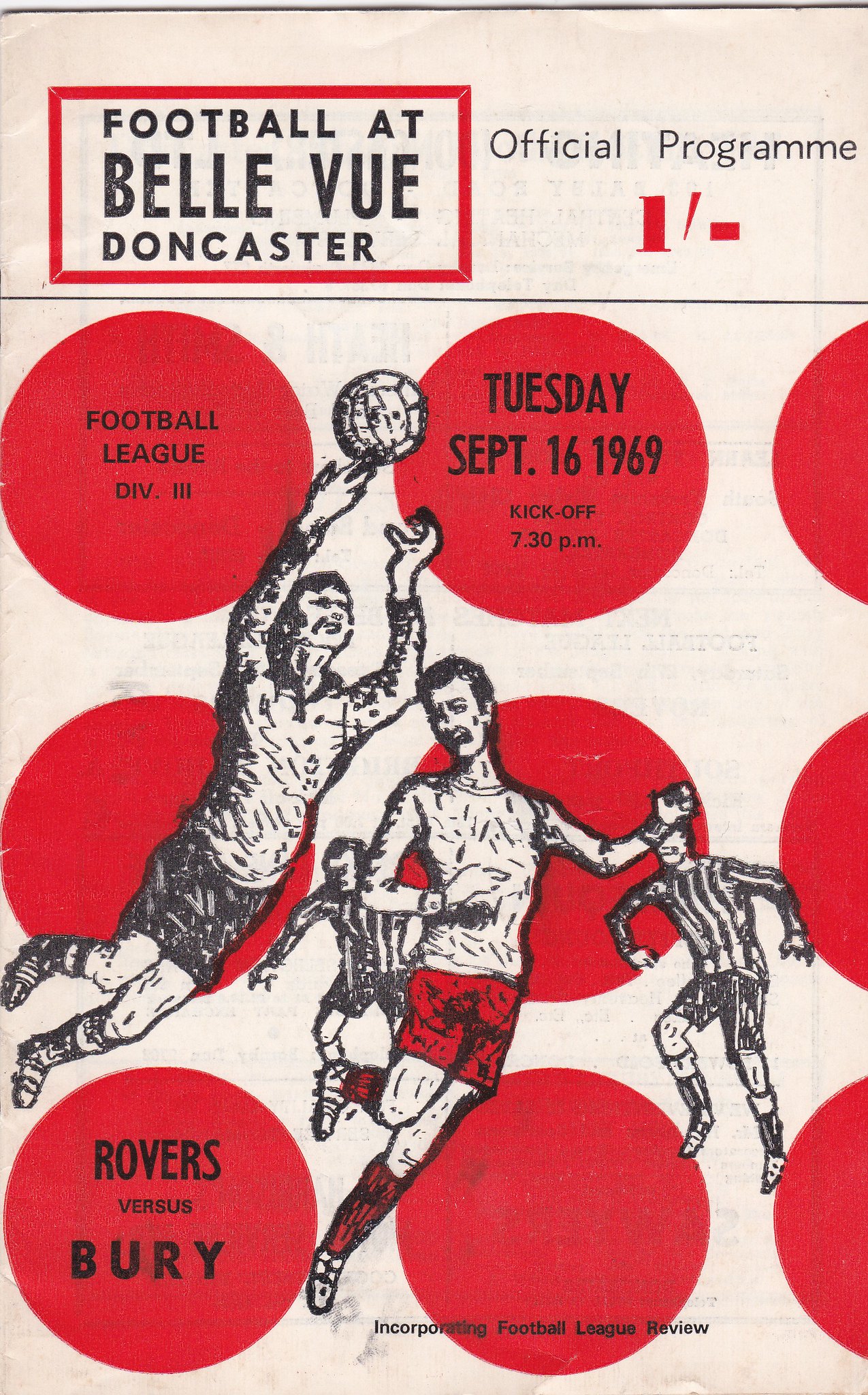This image is of a vintage football (soccer) program cover. At the very top, against a red square background, it features the title "Football at Bellevue Doncaster." To the right, it reads "Official Program 1-". The design incorporates whimsical, cartoonish illustrations of players in action. One player is shown leaping to catch a ball while another, possibly a teammate in red shorts and socks, stands by. In the background, there are two goalkeepers dressed in black and white striped jerseys. Below the illustrations, there are several footballs each containing text: one says "Football League Division 3," another details the event date "Tuesday September 16th 1969," with a kickoff time of 7:30 p.m., and the last ball on the bottom left states "Rovers vs. Bury." At the very bottom of the program, the words "Incorporating Football League Review" are printed. The overall design is described as unique and fun, scattered with polka dots and dynamic drawings of soccer players.